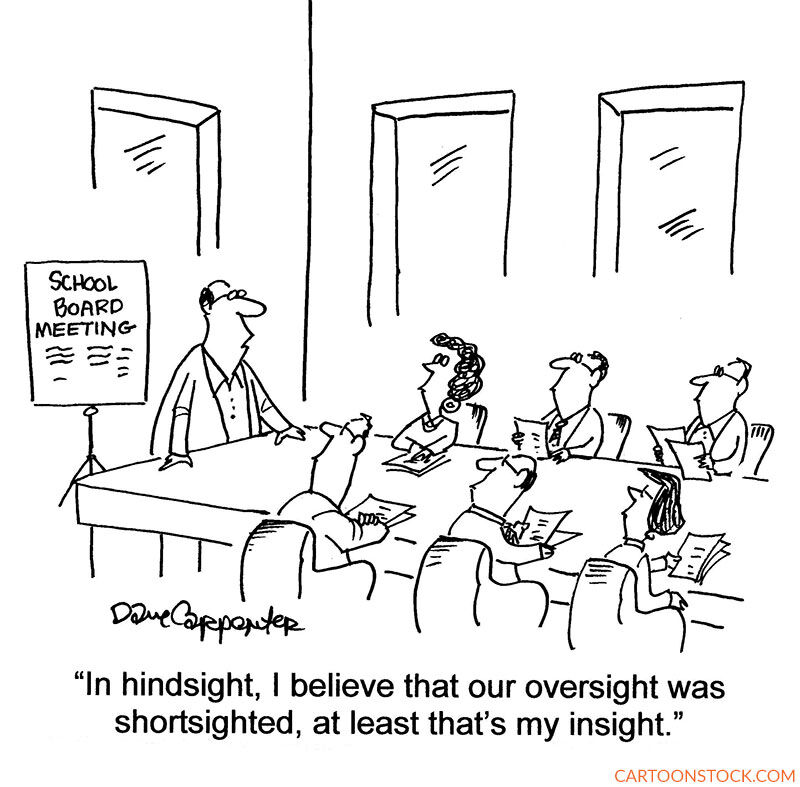This detailed black and white line drawing is a cartoon illustration by artist Dave Carpenter, identifiable by his signature beneath the drawing, above the caption. The scene captures a school board meeting, with a man in spectacles standing at the head of a boardroom table. He addresses six individuals seated around the table, each holding papers, and all attentively looking at him. The attendees consist of three women and three men, all wearing glasses. Behind the standing man, a poster reads "SCHOOL BOARD MEETING" in capital letters. The caption below humorously states, "In hindsight, I believe that our oversight was short-sighted. At least that's my insight." The background includes three unadorned windows. The image, characterized by sharp and precise lines, is predominantly black and white, save for the website address "CARTOONSTOCK.COM" written in orange, located in the lower right-hand corner.